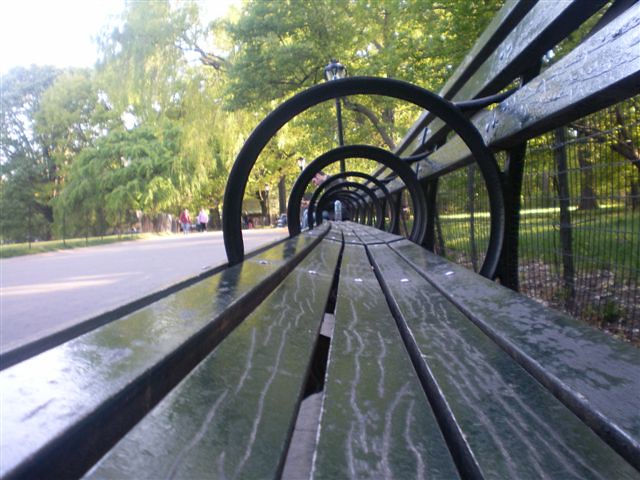This captivating park scene, likely in Central Park, features a park bench with distinctive anti-homeless bars that create a visually engaging tunnel effect. The photograph is taken on a bright, sunny day, with the camera positioned to look through the circular armrests of the park bench. The view extends through approximately six other benches lined up in a row, each with five greenish-gray wooden slats. 

The tunnel-like composition of black, round armrests grows smaller towards the distance, drawing the eye deeper into the image. Behind the bench, a black metal fence and a lush line of green trees are seen. To the right of the bench is a little gray road, with a stripe of green grass halfway along the page. Further behind the scene, there's a huge walkway and more vibrant greenery, along with a noticeable street lamp at the far end of the bench. A small building peeks out from the background against a bright, clear sky, completing this quintessential park depiction.